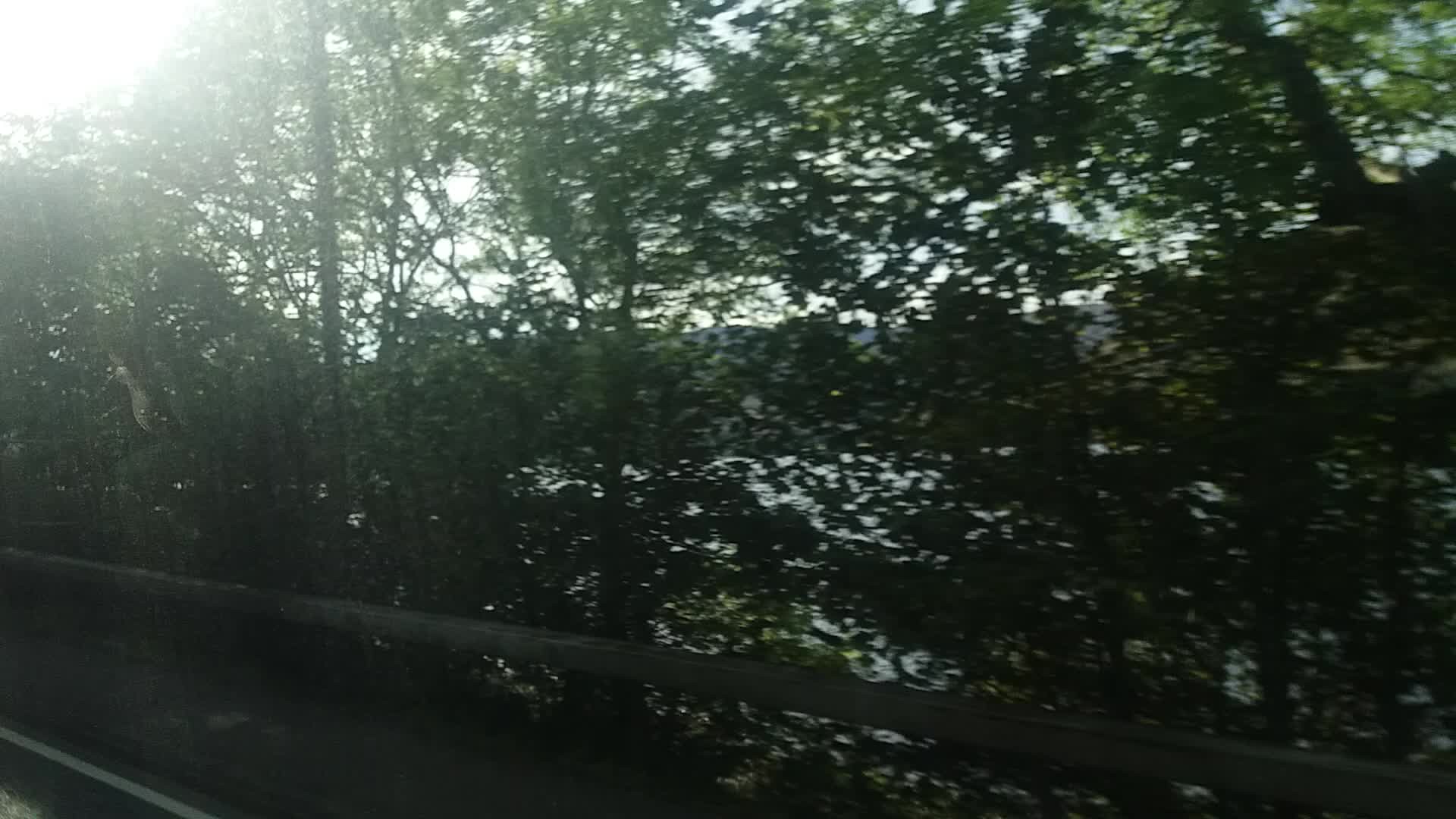A scenic view captures a serene moment on a lakeside road. In the foreground, a stretch of the road is visible, complete with the protective side rail and a sliver of the white line marking its edge. The road's proximity to the lake is highlighted as the water nearly meets the pavement. Interspersed among the dense grove of green-leaved trees, which line both sides of the road, are glimpses of a tranquil, expansive lake. The clear blue sky above casts a gentle glow, punctuated by sunbeams filtering through the canopy. Across the water, an additional row of trees along with distant hills enhances the picturesque landscape, complementing the calm and beauty of this natural setting.